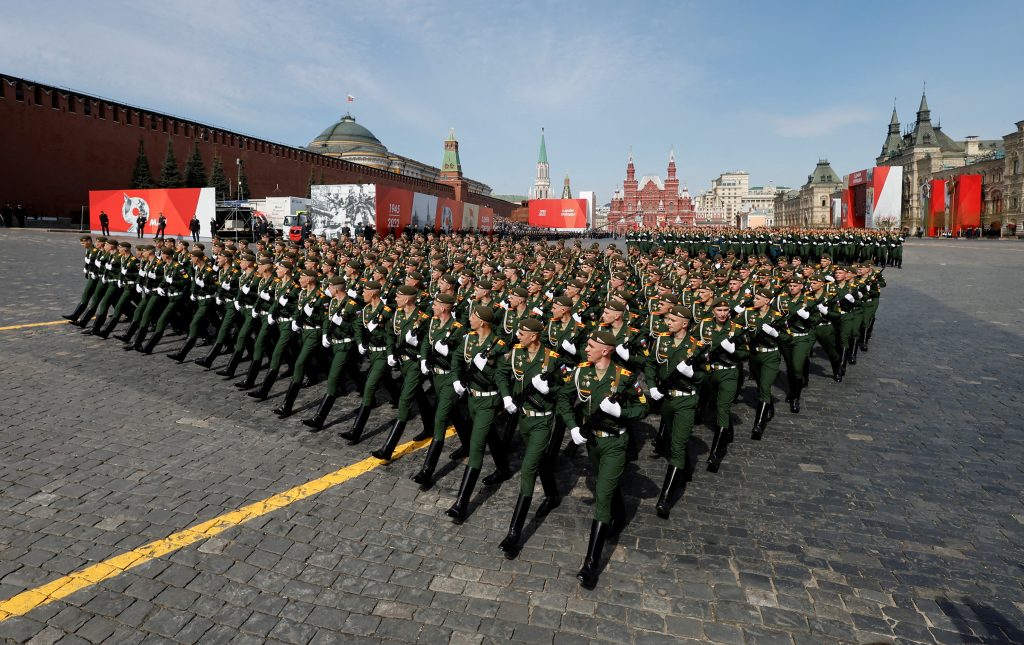The image depicts a meticulously organized military parade taking place on a bustling cobblestone city street, likely in a European country possibly resembling Budapest. The scene features rows of over 100 soldiers, all white males, clad in solid army green uniforms, adorned with white gloves, and beret-style brown hats. They are uniformly equipped with rifles held over their left shoulders and are marching in perfect unison, each with their left foot forward. Their tall, shiny black boots almost reach their knees, adding to the disciplined appearance as they step forward in sync.

The street itself is paved with cobblestones and has a yellow stripe down the middle, emphasizing its urban setting. The soldiers are arranged in large rectangular formations, with small spaces separating the groups, suggesting a grand display of military precision.

In the background, majestic, old-style buildings reminiscent of castles tower over the scene, reinforcing the European ambiance. To the left, a dome-shaped building painted green and white stands out among the structures, while another castle-like edifice and other significant architecture frame the surroundings. Red and white posters scattered along the street hint at an event being commemorated, though their inscriptions remain indistinct. The combination of the soldiers’ unwavering focus and the historical architecture creates a powerful and evocative depiction of the parade.